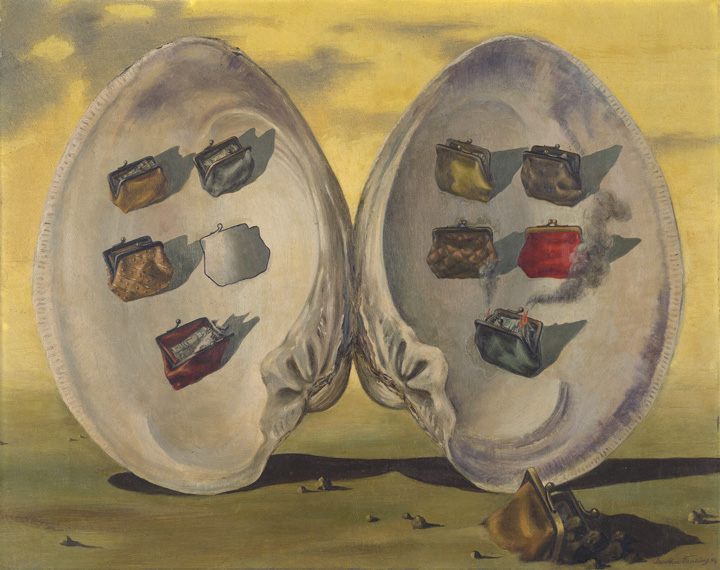The painting features an oversized white oyster shell standing upright and split open, facing the viewer against a surrealist backdrop of a moody yellow sky streaked with dark blue-gray clouds. The ground beneath the shell is a mix of green hues and scattered with small rocks. Inside the shell, the exposed interiors are shaded with touches of black and are adorned with a total of ten colorful coin purses on either side, arranged systematically across three rows. 

On the left half of the shell, there are five bags: starting from the top, gold on the left side and green on the right; the second row has yellow on the left and silver on the right; and at the bottom, there is a single red bag. These bags are all open, and at least three show visible money inside. There is also an empty outline where another bag might be.

On the right half, another five bags are positioned: gold, black, silver, red, and gray. While three of them remain open with two showing money inside, the others are closed. Notably, the bottom bag appears to be aflame, emitting small flames and black smoke.

In front of the shell, resting partially in the sand, lies an additional open bag. Something seemingly spills from it, potentially resembling rocks or even ducklings, adding an element of mystery to the composition.